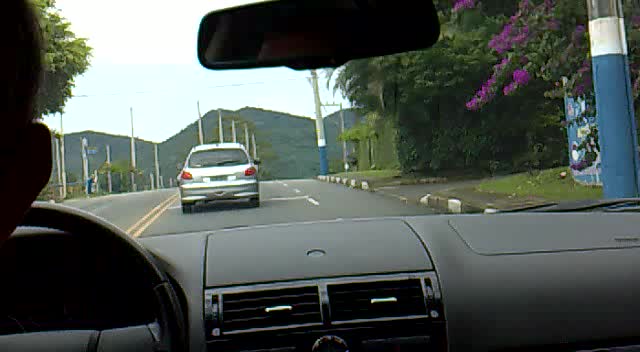This photograph captures a moment from inside a moving vehicle, taken from the middle of the back seat. Dominating the lower portion of the image is a black dashboard, with a glimpse of the black steering wheel visible at the bottom left. The dashboard itself is mostly unadorned and vacant of any visible instruments. On the top left of the image is the silhouette of a person, possibly a man with short hair, partially visible from behind. Above, towards the center of the frame, a black rear-view mirror is mounted. Below it, air vents are discernible in the middle of the dashboard, featuring small silver rectangular adjusters.

Outside the vehicle, a silver car can be seen ahead, driving on the right-hand side of the road. The left side of the road is marked by a yellow dividing line. On the right side of the frame, a white pole stands next to some green bushes and vegetation, signifying the roadside area. You can also make out the edge of a narrow sidewalk, though it is not prominent. Further in the background, a range of mountains stretches across the horizon under a clear, bright blue sky, indicating good weather conditions.